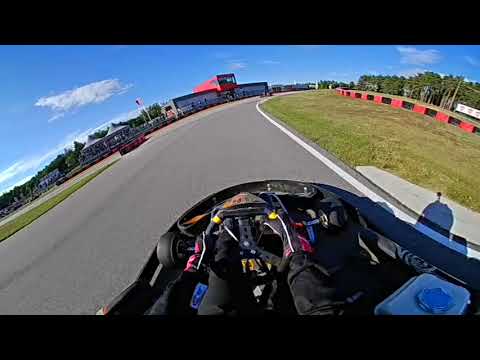This image captures an outdoor go-kart racing scene on a clear, sunny day with a blue sky and a few fluffy white clouds. The photo is taken from the viewpoint of a go-kart racer, showing an inside look at the black steering wheel adorned with yellow markings, gripped by the driver's hands in red gloves. The driver, sporting a black long-sleeve jacket and black pants, is navigating the dark gray track, which is bordered by solid white lines. 

Surrounding the track, the environment is lush and green, featuring grassy areas and trees, with a thin, red and black-marked barrier or fence running down the middle of the grassy infield. To the left of the track, there is a series of buildings, some of which have white canopies, and one building appears to be red, white, and blue. Farther off in the distance, there might be another vehicle in sight. 

A clear view of the controls inside the go-kart showcases the colored buttons and the white gas tank with a silver lid. The image exudes the excitement of go-kart racing under perfect weather conditions, accentuated by faint traces of spectators' galleries positioned along the left side of the track.